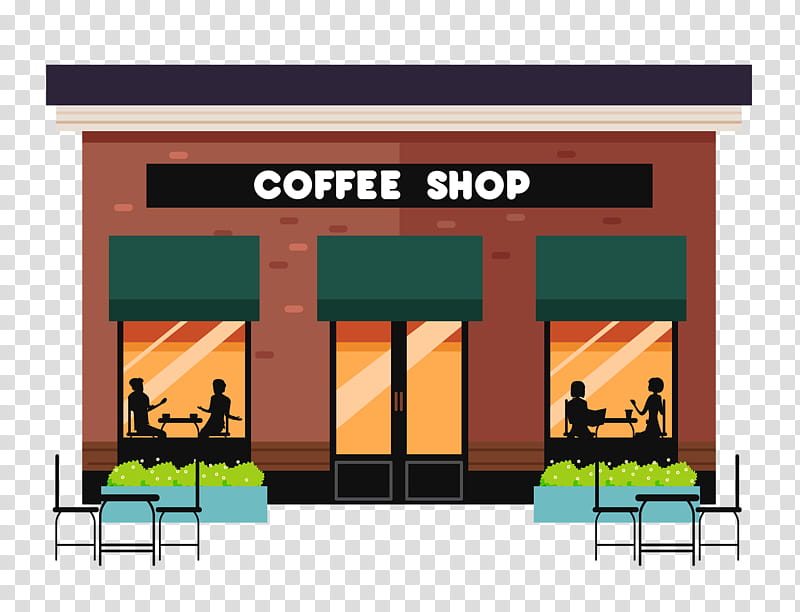The image features a computer-generated, cartoony rendering of a coffee shop set against a background of gray and white checkered transparency. The coffee shop, rectangular in shape, is constructed with brownish bricks and topped with a black roof that has a white underside. Prominently displayed on a black rectangular sign at the top center of the building are the words "Coffee Shop" in white lettering.

The façade includes a pair of windows with orange-tinted glass and a central set of double glass doors. Each window is adorned with green awnings. Reflective glares on the windows showcase the creator's attention to detail, emphasizing the glassy texture. Silhouettes of two people are visible in each window, seated at tables with coffee cups in front of them, against a background of yellow wallpaper with light brown or blue trim.

Adding to the charm, the coffee shop is surrounded by light brown rectangular flower boxes, filled with greenery and yellow or white flowers. These planters sit beneath the windows, flanking two black circular patio tables with matching chairs. This inviting outdoor seating area completes the quaint and inviting scene.